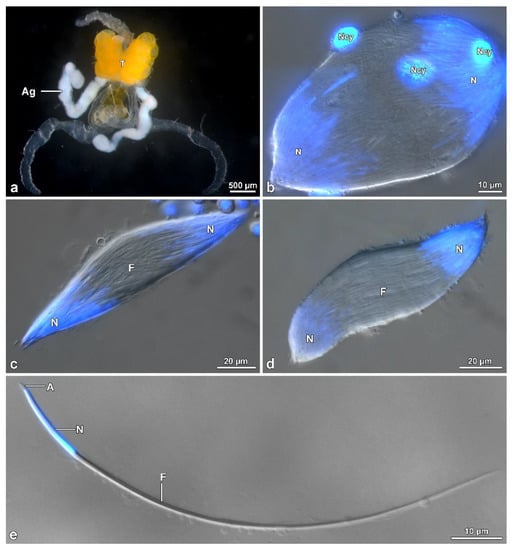The set comprises five microscopic images displayed on a black background. 

Top left (Image A): A dark microscope slide showing an orange, almost bell pepper-shaped top with two white squiggles emerging from it. Below the orange part, a transparent gray cone extends, further connected to two gray squiggles. The white text "AG" labels one of the white squiggles, and a lowercase 'a' is marked in the bottom left corner. The slide is labeled "500 p.m.".

Top right (Image B): A slightly deflated, oval-shaped figure with blue edges on the bottom left and top right, a black center, and a lowercase 'b' in the bottom left corner. This image is noted as "10 p.m.".

Middle left (Image C): An image similar to B but more elongated with sharper oval ends. It displays a combination of gray, white, and blue colors with a 'c' in the bottom left corner and labeled "20 p.m.".

Middle right (Image D): Another variation of the elongated figure, appearing fatter and labeled 'D'.

Bottom (Image E): A large rectangular image featuring a singular curved strand that begins in bright blue at the top left and transitions to dull gray. The gray color extends like fluid filling a space. It carries a lowercase ‘e’ in the bottom left corner.

Each successive image presents a progressively altered view of the same basic structure, reflecting different magnifications or states.